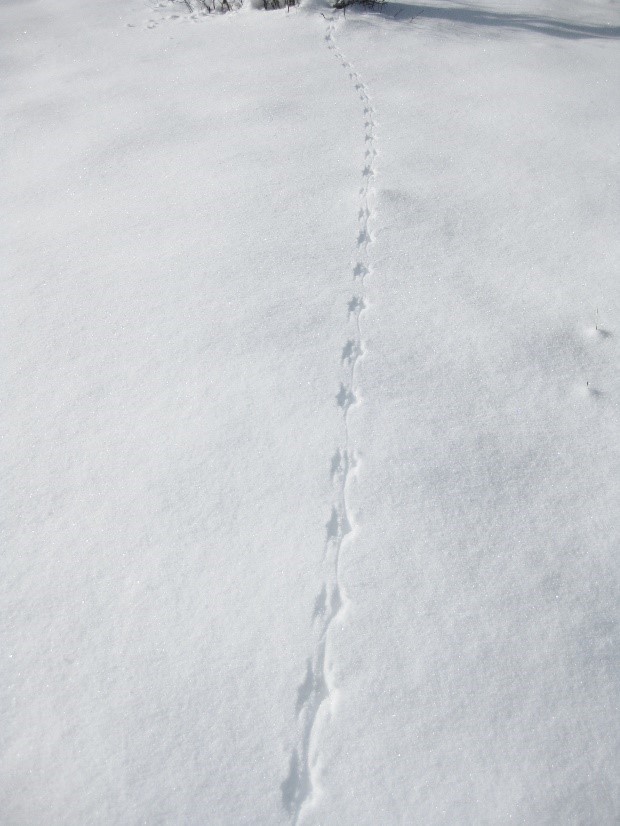This vertically oriented outdoor photograph, taken in winter, captures a serene, snowy landscape. The pristine, smooth, white snow stretches uninterrupted across the rectangular frame. The main subject of the photo is a continuous track that starts from the bottom and meanders slightly before curving at the top. These tracks, numbering around 20, appear to be created by a small animal with closely spaced feet, possibly a rabbit or a bird. The trail, indicative of hopping, extends from the foreground to the background, suggesting the animal's journey. Adding context to the scene, a shadow cast in the upper right corner hints at the presence of a bush or small branches, and the late evening sunlight creates a tranquil, wintry ambiance.